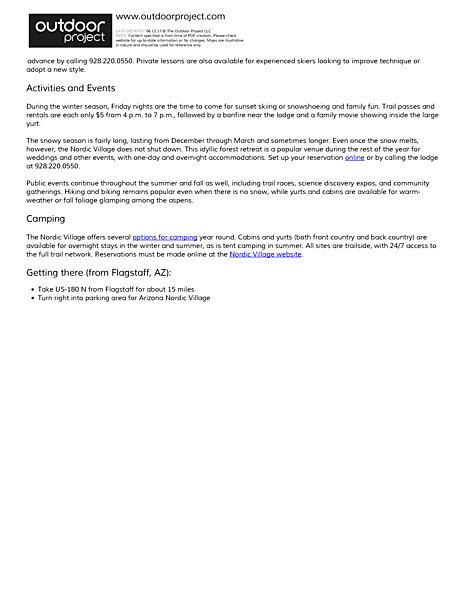The screenshot captures an image featuring detailed information about the Arizona Nordic Village, a year-round destination for outdoor enthusiasts. At the top, the header consists of a black rectangle with "Outdoor Project" written in all lowercase white letters, followed by the URL www.outdoorproject.com. Below the website address, there is some text that is too small and blurry to decipher.

The main content of the image provides extensive details about the activities and services offered by the Arizona Nordic Village. It begins with a contact number, 928-220-0550, for making advance reservations. It also mentions that private lessons are available for experienced skiers to refine their techniques or learn a new style.

During the winter season, Friday nights are highlighted as prime times for sunset skiing or snowshoeing and family fun. From 4 p.m. to 7 p.m., trail passes and rentals are priced at just $5. These evenings conclude with a bonfire near the lodge and a family movie showing inside a large yurt. The snowy season typically extends from December through March, though it can last longer depending on conditions.

Even after the snow melts, the Nordic village remains a popular destination. It serves as a venue for weddings and other events, offering both one-day and overnight accommodations. Reservations can be made online or by calling the lodge at 928-220-0550. Public events continue throughout the summer and fall, including trail races, science discovery expos, and community gatherings. Hiking and biking are popular activities in the warmer months, with yurts and cabins available for glamping among the aspens.

For camping enthusiasts, the Nordic village provides year-round options. Cabins and yurts, available in both front country and backcountry settings, can be booked for overnight stays in both winter and summer. Tent camping is also available during the summer months. All camping sites are conveniently trail-side with 24/7 access to the full trail network. Reservations must be made online via the Nordic village website.

To get to the Arizona Nordic Village from Flagstaff, Arizona, take US-180N for approximately 15 miles, then turn right into the parking area for the Arizona Nordic Village.